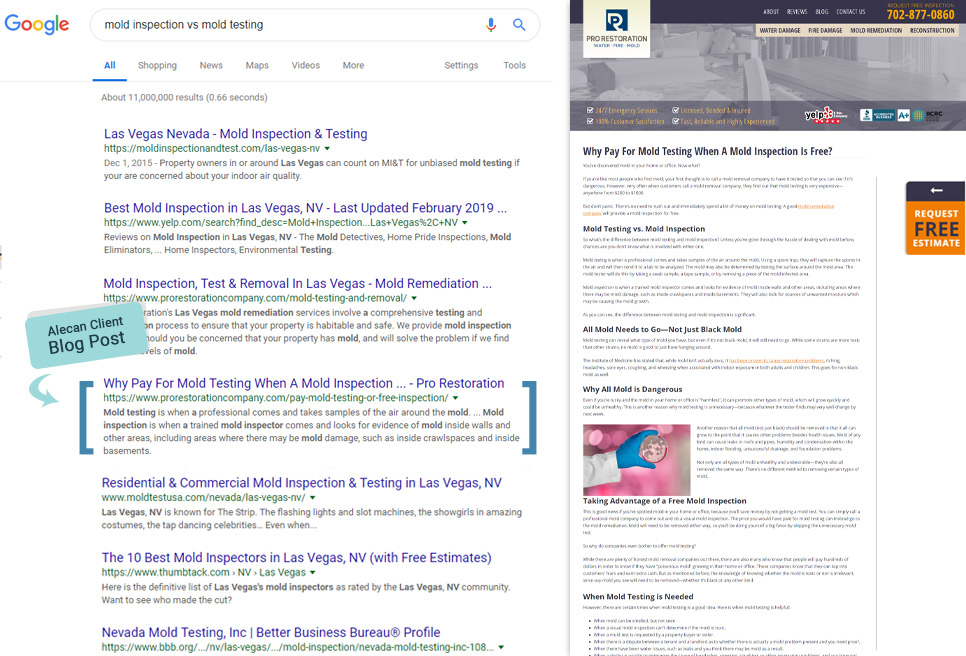The image features a split-screen view displaying two different pages side by side. On the left-hand side, a Google search query for "mold inspection versus mold testing" is shown, revealing seven search results. The fourth search result, highlighted in blue brackets, is a link to a website called ProRestoration. The title of that link reads, "Why pay for mold testing when a mold inspection…" and is truncated. An informational pop-up accompanies this result, prompting the viewer to "allocand client blog post here."

On the right-hand side of the screen, the corresponding blog post from ProRestorationCompany.com is displayed. The URL for this blog post is detailed and reads: ProRestorationCompany.com/pay-mold-testing-or-free-inspection. The headline of the blog post matches the search result: "Why pay for mold testing when a mold inspection is free." The page contains an extensive text explaining the topic in detail.